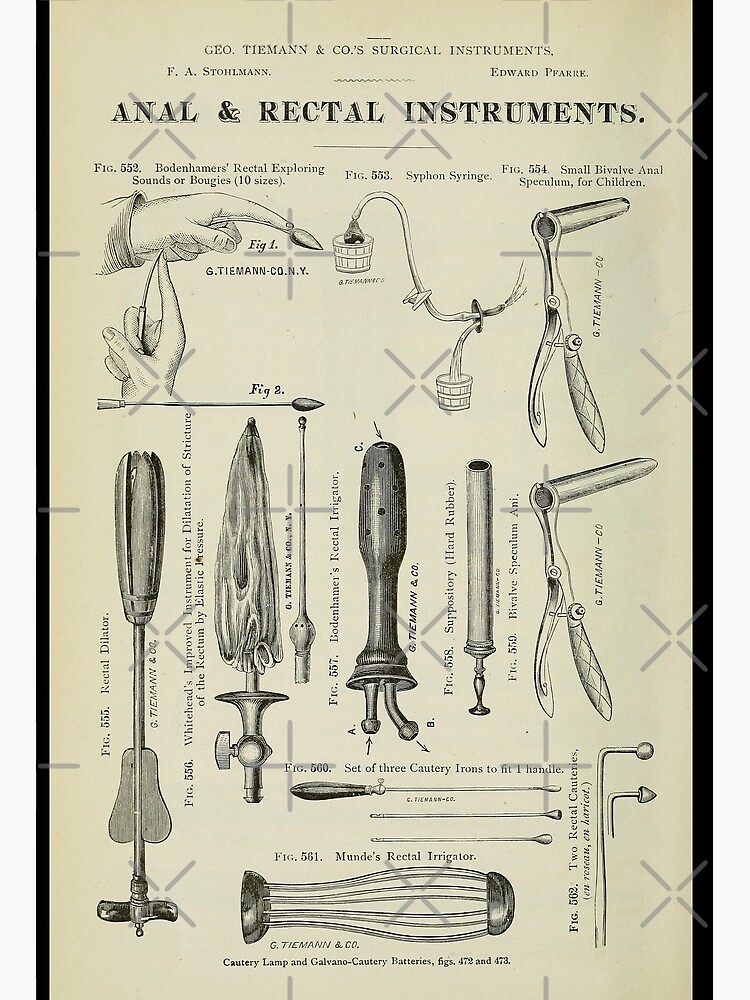This black and white medical illustration, set against a slightly tan background, is a detailed display of various surgical instruments specifically designed for anal and rectal procedures. The title at the top reads "George Tiemann and Co's Surgical Instruments" with the names "F.A. Stolman" and "Edward Peer" mentioned below. The large, prominent title announces "Anal and Rectal Instruments." The instruments are labeled with specific figures and descriptions:

- "Figure 552, Bowden Hammers, Rectal Exploring Sounds, or Bougies, 10 sizes" shows a finger with a probe attached to its end.
- "Figure 553, Siphon Syringe" features two buckets connected by hoses to another instrument.
- "Figure 554, Small Bivalve Anal Speculum for Children," which has a handle, tube, and an adjustable screw.

The illustration includes images of various other instruments: a plier-like device with rounded tops, a whisk-like instrument, and several different speculums and rectal dilators. Additional textual elements are present but not fully legible. Throughout the illustration, there is a white watermark with a drop shadow that reads "Curb Digger Carl." This detailed drawing captures the diverse range of surgical tools used in historical anal and rectal medical procedures, each meticulously labeled and depicted.